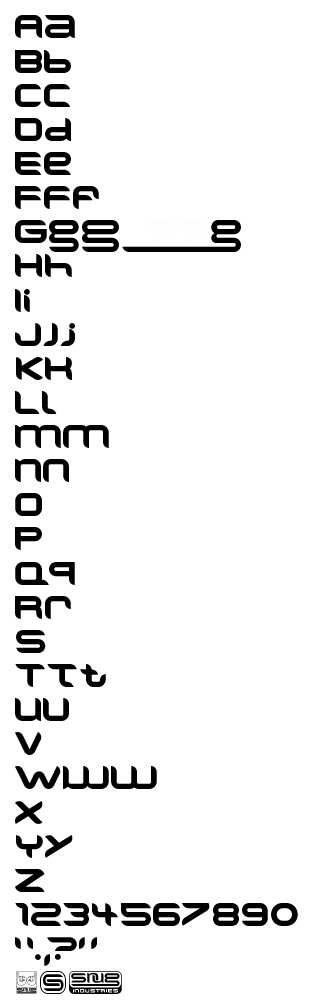This vertical image showcases an extensive display of various fonts and characters, primarily focusing on the alphabet. The sequence begins with the letter "A," pairing both its capital and lowercase forms. This pattern persists throughout the alphabet until the letter "F," which unusually features three variations of the letter "F" aligned horizontally.

Unique characteristics appear with the letter "G," where a standard capital G is accompanied by two larger, script-styled lowercase Gs. A notable long line separates another G that extends further to the right, creating an unusual alignment. Some letters, such as "K," appear to possess stylistic differences suggesting they might belong to foreign scripts, though this isn't definitively clear.

Intriguingly, the alphabet progresses with both letters "M" and "N" presented solely in lowercase. Other letters such as "O," "P," and "S" have only single representations, whereas elsewhere multiple depictions exist. For example, the letter "T" appears three times: a standard capital T, a capital T with an extended right stroke at the base, and a lowercase script T with its tail looping upward to the right.

The "W" character also appears thrice: a standard W, one with a small tail, and another with a more rounded shape. This diversity in portrayal introduces ambiguity about whether these variations are due to differing fonts or representative of different languages.

Beneath the alphabetical array are numerals, listing from "1" to "9" followed by "0." Further below, an assortment of punctuation marks is included. Concluding the image are several logos, arrayed at the bottom, subtly grounding the eclectic typographical showcase.